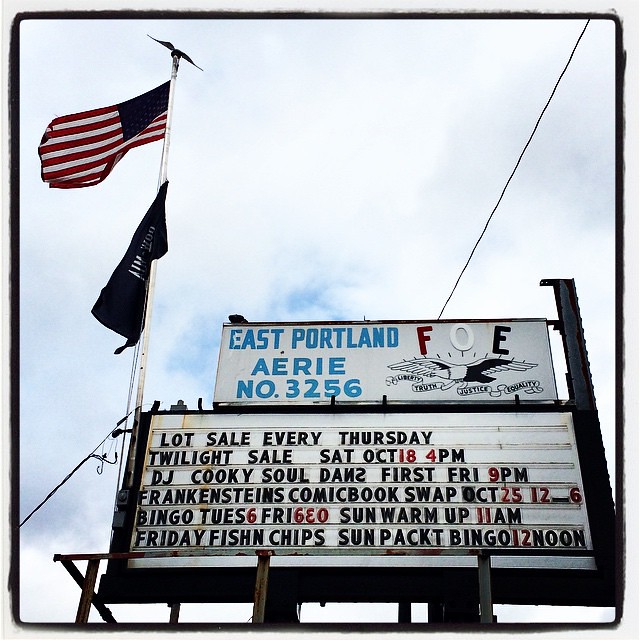This detailed color photograph, presented in a square format, captures an upward view of a large billboard-style sign set against a backdrop of a mostly cloudy blue sky. The scene prominently features a flagpole on the left-hand side, adorned with the American flag at the top, and a folded, black flag beneath it. At the top of the billboard on the right, a banner reads "East Portland FOE Aerie No. 3256" in blue letters, flanked by a black and white eagle emblem with "FOE" displayed in red, white, and blue lettering. The central portion of the sign consists of a white marquee with changeable black magnetic letters, advertising local events: "Lot Sale every Thursday," "Twilight Sale Saturday October 18 4 p.m.," "DJ Cookie Soul Dance First Friday 9 p.m.," "Frankenstein's Comic Book Swap October 25th from 12 to 6," "Bingo Tuesday 6, Friday 6:30, Sun Warm-Up 11 a.m.," and "Friday Fish and Chips Sunday Packet Bingo 12 noon." This sign, mounted on a sturdy black metal structure, stands tall with power lines running overhead, providing a snapshot of vibrant community activity.